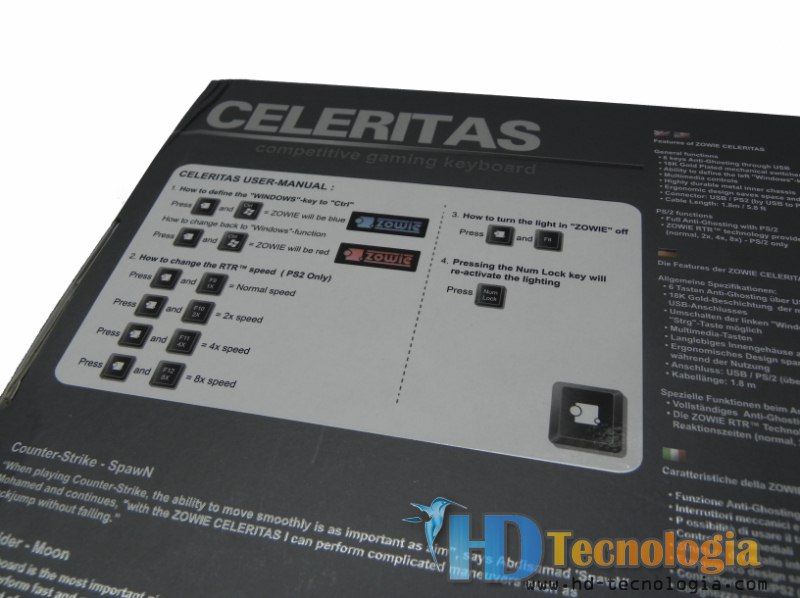The image displays a close-up of a black box for the Celeritas competitive gaming keyboard. The front of the box features the title "Celeritas Competitive Gaming Keyboard," along with essential instructions. Centrally placed on the box is a silver diagram, designed to serve as a user manual. This diagram illustrates how to redefine the Windows key to Control and adjust the RTR speed, which is specific to PS2 connection, offering options for normal, 2x, 4x, and 8x speeds. Additionally, it explains how to turn the Zowie lighting on or off by explaining the combination of key presses needed. The Zowie indicator light changes color based on function: it turns blue when the Windows key is redefined as Control and red when reverted back to the Windows function. The layout of the instructions consists of a series of icons and formulas, making it complex to read from the angle of the photo. In the bottom right corner, the logo and the words "HD Technologia" are prominently displayed, with "HD" in blue and "Technologia" in yellow. Also noticeable is a blue hummingbird graphic situated over the black background. Multiple language translations are scattered around the box, ensuring a broad user comprehension.